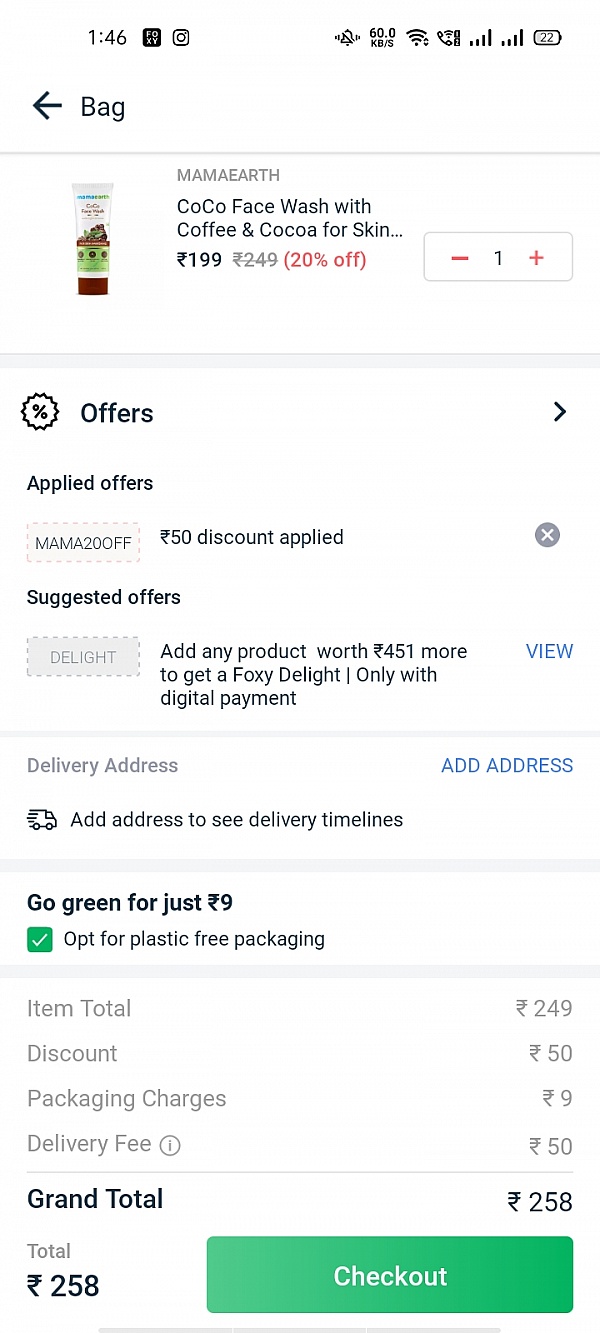Screenshot from an online retailer app showing a customer's basket. The basket contains one item: a cocoa face wash with coffee and cocoa from Mama Earth, priced at 199 units of currency. The customer has applied the promo code "MAMA20OFF," which grants a discount of 50 currency units. An additional 9 currency units have been charged for plastic-free packaging, and a delivery fee of 50 currency units has been added. The total cost amounts to 258 currency units. The customer has yet to enter a delivery address.